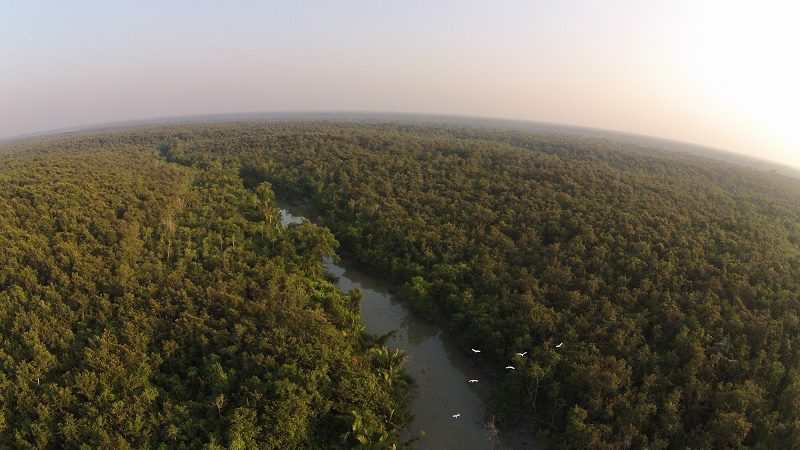This aerial photograph showcases a breathtaking forested landscape taken from a high vantage point, revealing a vividly detailed scene. The image is dominated by a dense canopy of dark green trees that stretches across the entire frame, flanking both sides of a narrow, meandering river. The river begins at the bottom center of the image, curving gently leftward as it flows upward and eventually vanishing into the thick foliage just above the center. In the lower portion of the image, slightly right of center, there is a cluster of six white birds, either in flight or perched, appearing as tiny specks against the dark backdrop. The curved horizon, imparted by the camera lens, arcs slightly up from the left edge of the photo before dipping down towards the right, accentuating the depth and breadth of the landscape. The sky above the horizon transitions from a subtle orange glow near the horizon to a gradient of blue, with the upper left corner being blue-gray and the upper right corner glowing brightly, indicative of the sun situated just outside the frame to the right. This serene and untouched natural scene captures the wild beauty of the forest and river, unmarred by any man-made structures.